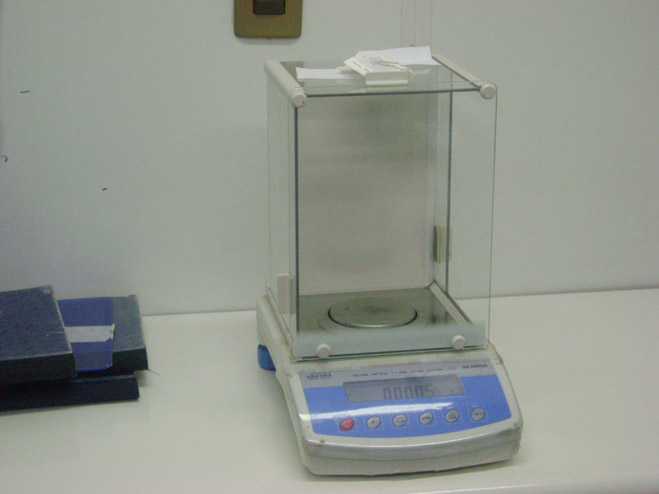The image depicts a piece of laboratory equipment, likely a weighing scale, situated on a white table against a white wall. The apparatus features a transparent cube glass container on top with gray or silver railings along its edges, allowing visibility inside. Below the container, the device consists of a blue and white scale. The scale's panel displays the reading "0005" on an LED screen and is encased in a gray or silver outer frame. The panel includes several buttons, five gray and one red, presumably for various functions like units of measure or power control. Additionally, there are folders or papers on the left side of the table.